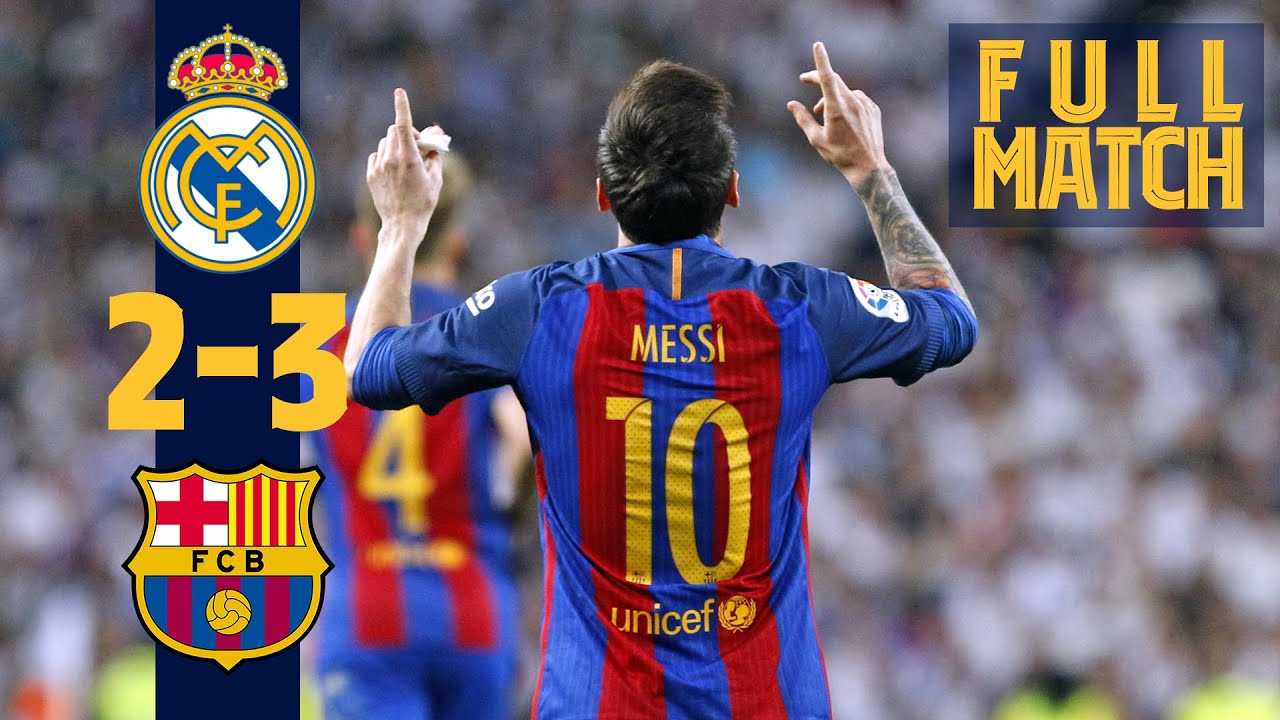The photograph is an advertisement for a full soccer match featuring the famous player, Messi. In the upper right-hand corner, large yellow capital letters read "FULL MATCH." Messi is central in the image, facing away from the photographer, dressed in a light blue jersey with blue and red stripes. His name "Messi" and number "10" are displayed prominently in yellow font on his back. His short brown hair is neatly parted to the side, revealing his light skin tone and a tattoo on his right arm. Messi's arms are raised with one finger pointing up, as he looks upward, seemingly towards the crowd, which appears as a blurred mix of red, white, and blue colors in the background. On the left side of the picture, two soccer team logos are displayed within a vertical navy blue rectangle. One logo features a crown and the letters C and F, while the other shows an FCB crest in black letters. Below these logos, the numbers "2-3" indicating some match statistics or score, are visible in yellow font.